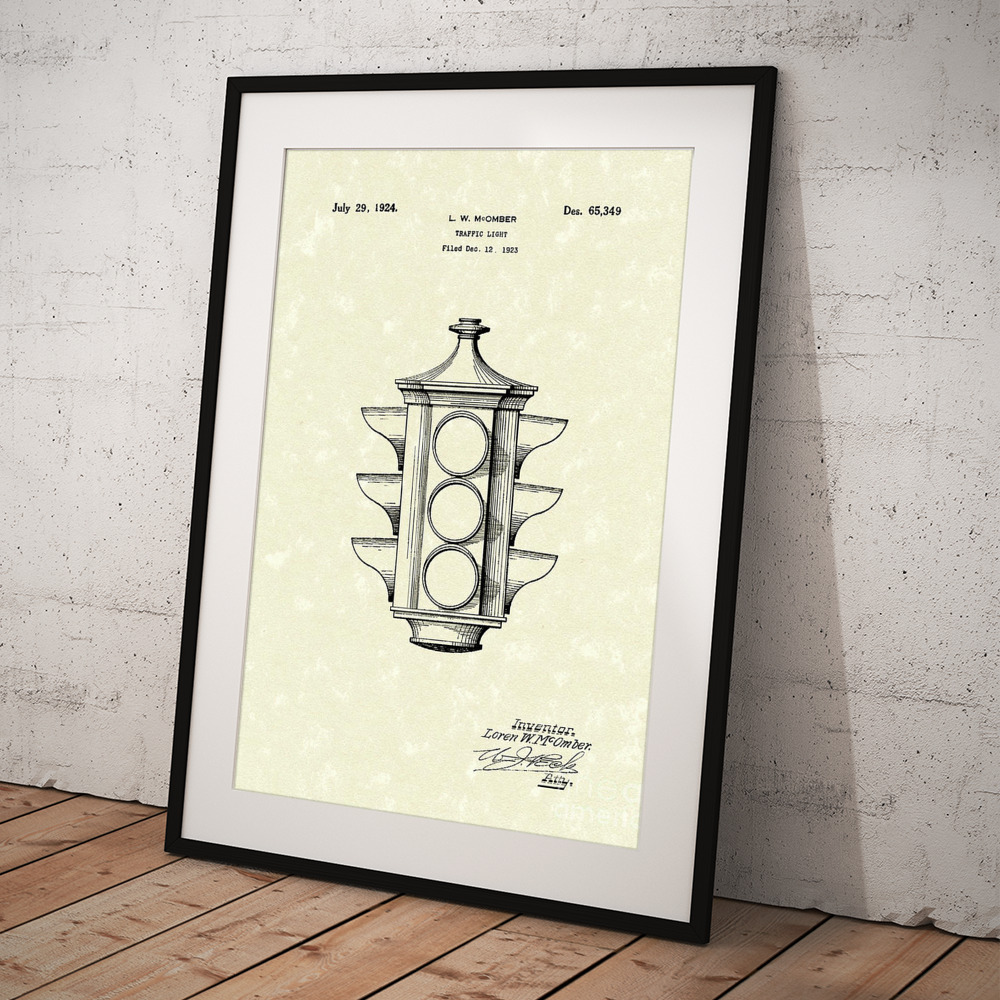The image is a detailed, black and white pencil drawing of a traffic light, showcasing three sides of the device. This illustration, dated July 29, 1924, appears on a parchment-like paper with text indicating "Traffic Light, filed December 12th, 1923" and the patent number "DES65,349" on the upper right. At the bottom right corner, it features the name of the inventor, Lauren W. McHumber, along with his signature. The drawing is encased in a thin black frame with white beveled edging, all set against a whitish plaster wall with small holes, resting on a wooden slatted floor. This framed artwork resembles a patent filing, preserving the historical significance of the traffic light's invention.